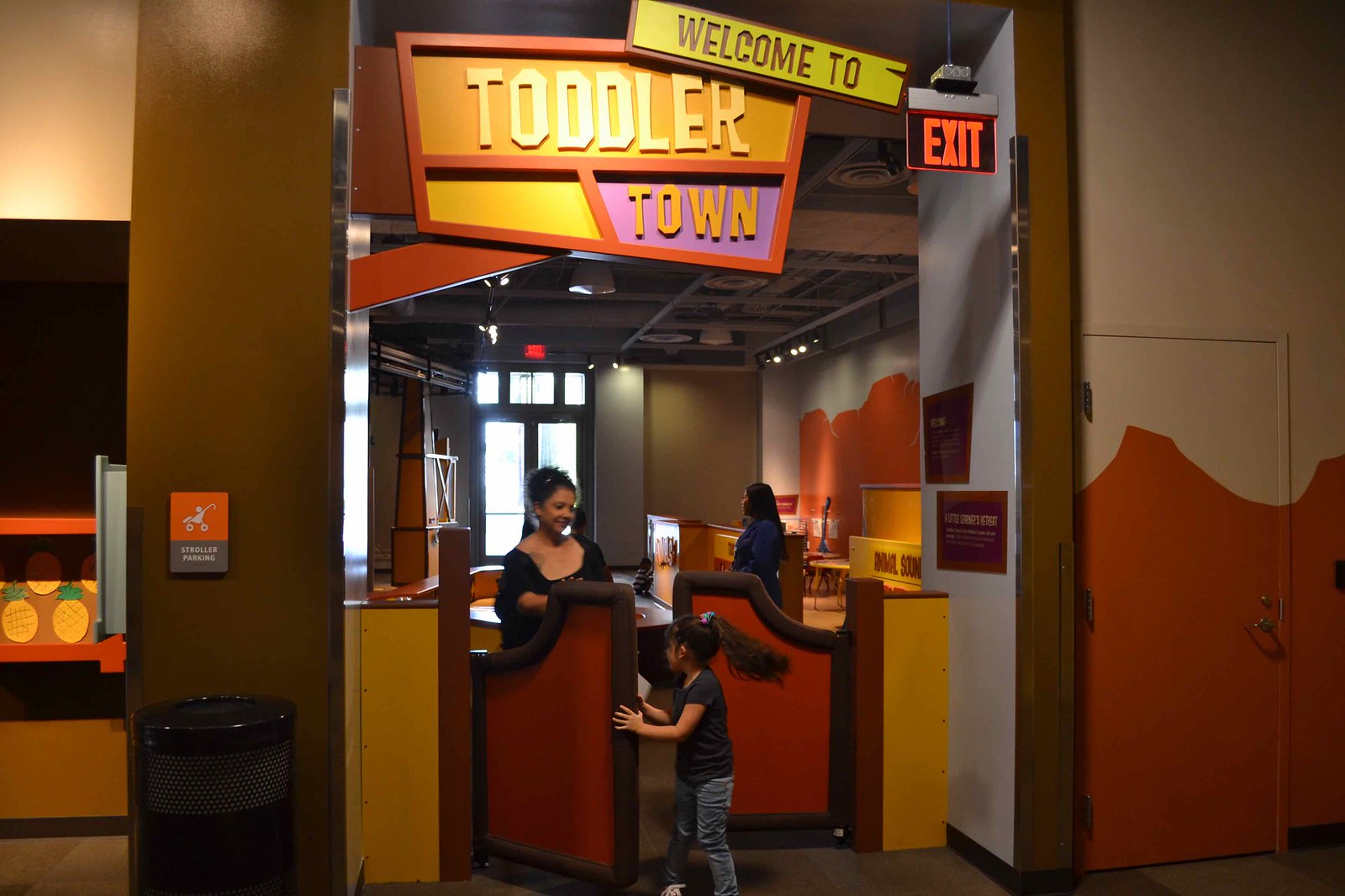The image captures the entryway to Toddler Town, prominently featuring a banner at the top that reads "Welcome to Toddler Town." An exit sign is also visible. As viewers approach the entrance, they note a wastebasket positioned on the left side. The right side of the entryway is adorned with walls painted in various colors, adding a vibrant touch.

A little girl is seen navigating through the swinging doors, holding one side open; it's unclear whether she is entering or exiting. She is greeted by a smiling woman who appears to be welcoming her. Within the establishment, another woman can be seen looking out over the interior of Toddler Town.

The scene is bathed in a cheerful palette of orange, yellow, and light blue hues. The environment suggests that Toddler Town might be a business, potentially a restaurant, with a small stage area on the right, possibly intended for performances or entertainment.